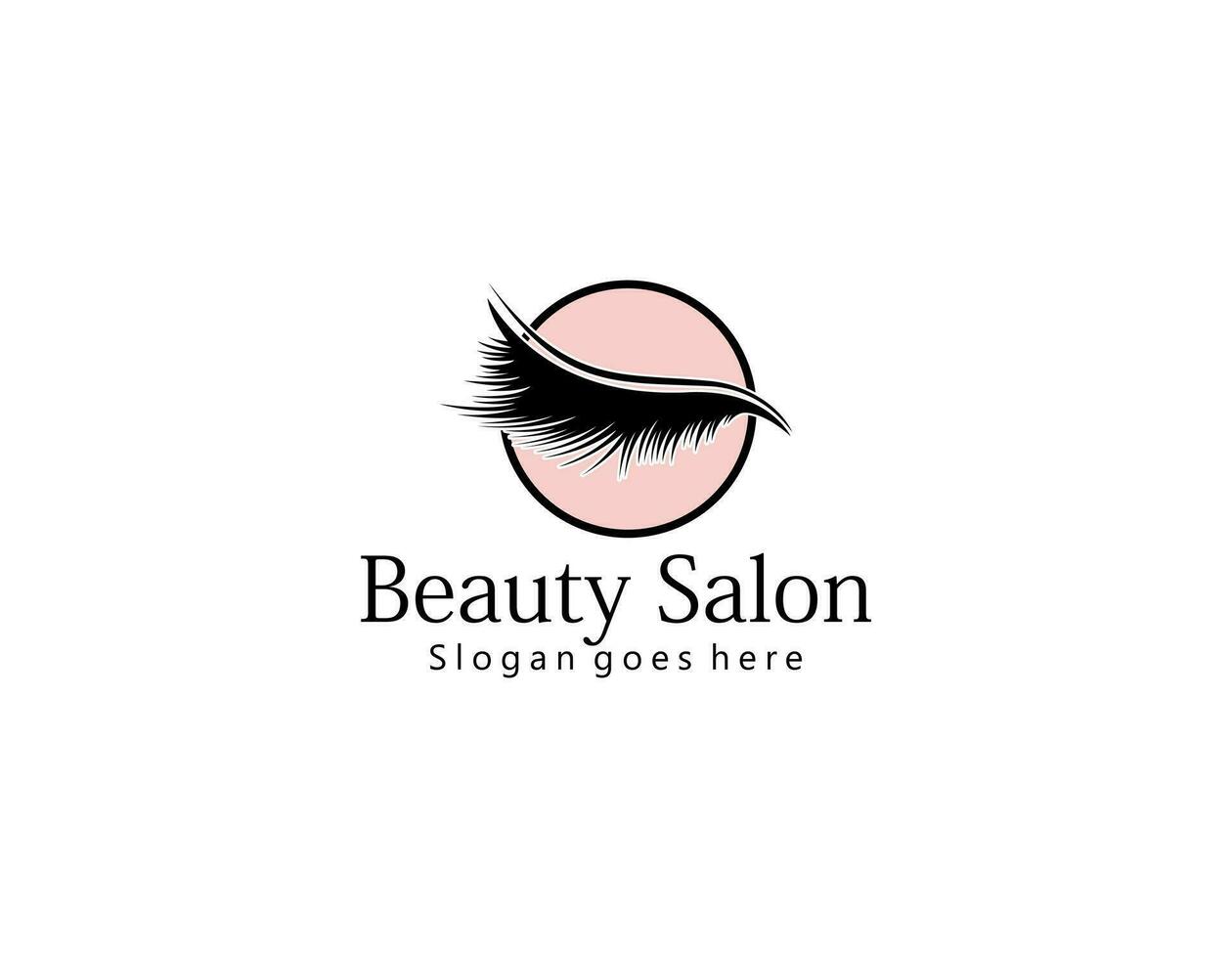The image is an example of a logo-style graphic set against a stark white backdrop. Central to this design is a circular logo, outlined in black and filled with a light pink, flesh-like color. The circle appears to represent a closed right eye, characterized by a striking black, wavy eyelash graphic that swoops downwards, suggesting fullness and individual black lashes, possibly indicating false eyelashes due to their fluffy and full appearance. Above the eye, delicate white tips edge the eyelashes. Beneath this detailed circular logo, the words "Beauty Salon" are displayed in black upper and lowercase lettering, with the phrase "slogan goes here" written under it. This sample image, ideal for signage or web page use, clearly showcases its intended use for a beauty salon.